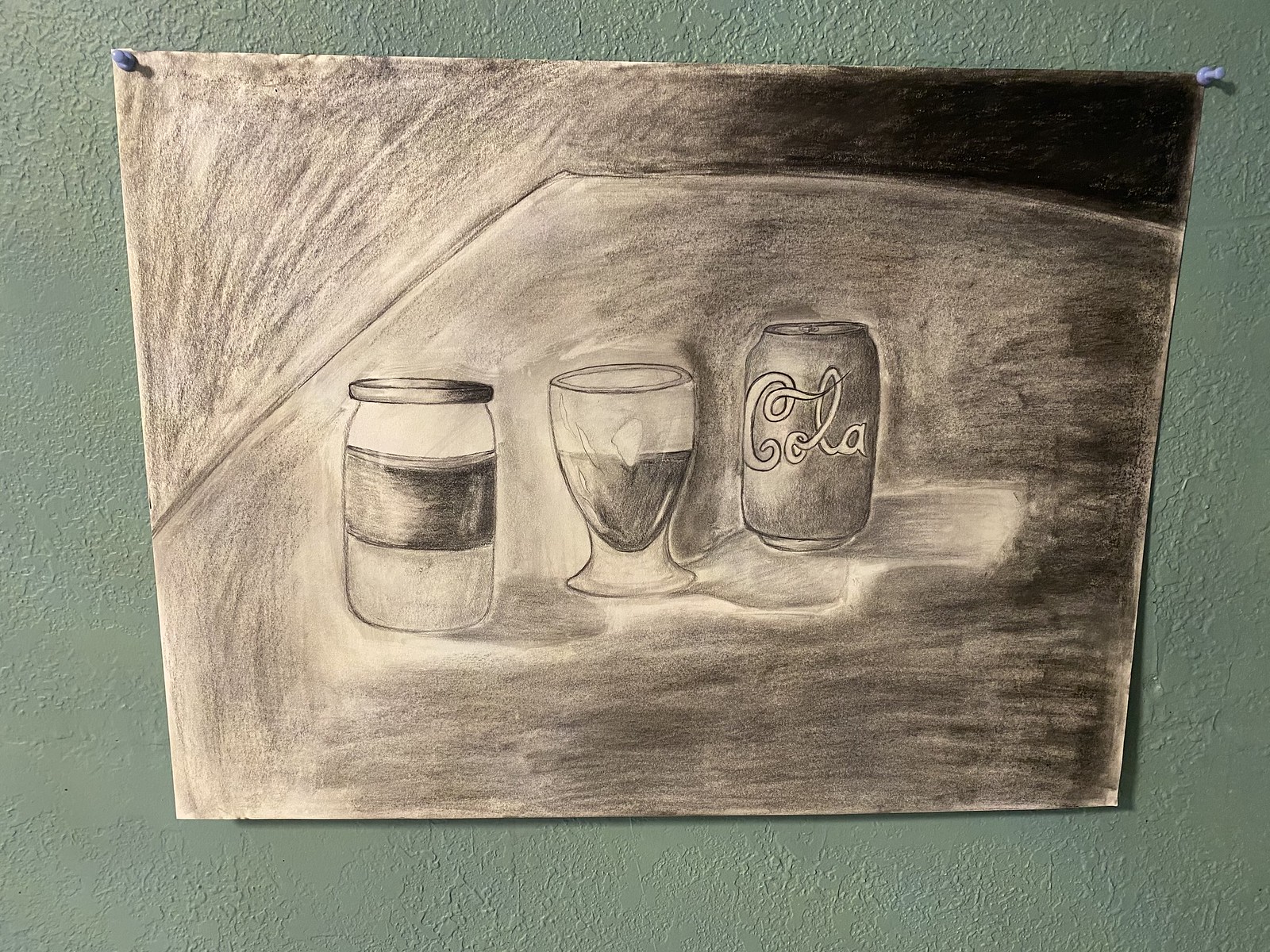In the photo, a light teal wall serves as the background, adorned with a piece of paper tacked up by two thumbtacks. The paper features a detailed sketch, likely drawn with colored pencils or charcoal, depicting a modest still life scene. On the left of the table in the sketch, an empty pickle jar with a lid and a label is prominently displayed. Beside the jar sits what appears to be a shot glass, and to the right, an aluminum can simply labeled "cola." The room is dimly lit, accentuating the intricate pencil strokes and giving the scene a somber, muted tone.